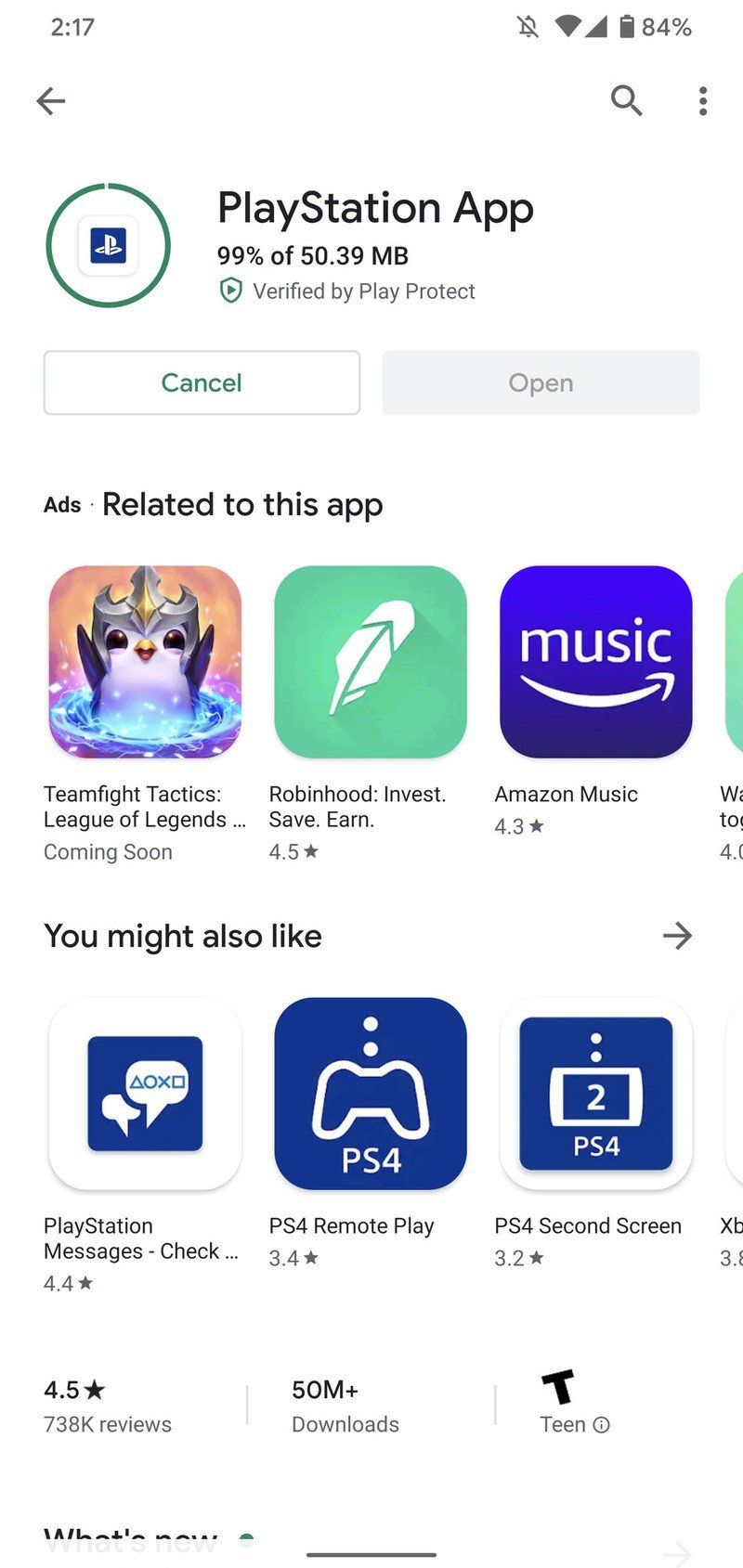The image displays the interface of a downloading app, specifically the PlayStation App, which is located at the top. The download progress bar shows it is 99% complete out of a total of 50.39 megabytes. Below the progress bar, there are two buttons: "Cancel" on the left and "Open" on the right, with the latter being grayed out, indicating it is not yet clickable.

Under these options is a section titled "Ads related to this app". The first advertisement promotes "Teamfight Tactics: League of Legends," marked as "Coming Soon." Next to this, there's an ad for "Robinhood: Invest, Save, Earn," followed by an ad for "Amazon Music" which is rated 4.3 stars.

Below the advertisement section, there is a row titled "You might also like." The first suggestion is "PlayStation Messages," followed by "PS4 Remote Play," and "PS4 Second Screen." Additional details include a 4.5-star rating for the PlayStation Messages app, over 50 million downloads for the PS4 Remote Play, and a "T-Teen" rating for the PS4 Second Screen app.